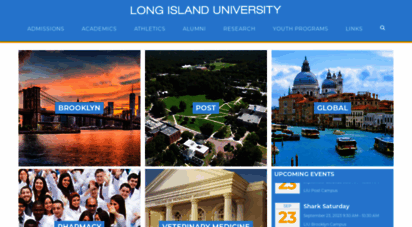The homepage of Long Island University’s website is displayed. The top section of the page features a light blue banner with the university's name, "LONG ISLAND UNIVERSITY," prominently centered in white capital letters. Below this banner is a white navigation menu with options that read, from left to right: Admissions, Academics, Athletics, Alumni, Research, Programs (partially obstructed), a partially readable option, and a search magnifying glass icon.

A yellow stripe is positioned beneath the navigation menu, while the rest of the content area is set against a white background. The website highlights various attributes of the university through a series of images:

- On the far left, there’s an image of the Brooklyn Bridge at sunset, labeled "Brooklyn" with a central blue button bearing the word "Brooklyn" in white text.
- To the right, an aerial view of a campus is showcased, labeled "Post" with a similar blue button in the center featuring white text reading "Post."
- Next, there is a picturesque scene of a canal in Venice, identifiable by its iconic blue-domed structure, marked "Global" with a central blue button displaying this label in white font.
- Below these images, there’s a partial photo featuring a group of doctors or pharmacists with the word "Pharmacy" partially visible.
- Adjacent to this is a substantial white building labeled with what seems to be "Veterinary Medicine."

On the right side of this section, there is a blue box labeled "Upcoming Events," completing the detailed overview of the university's key highlights and features.